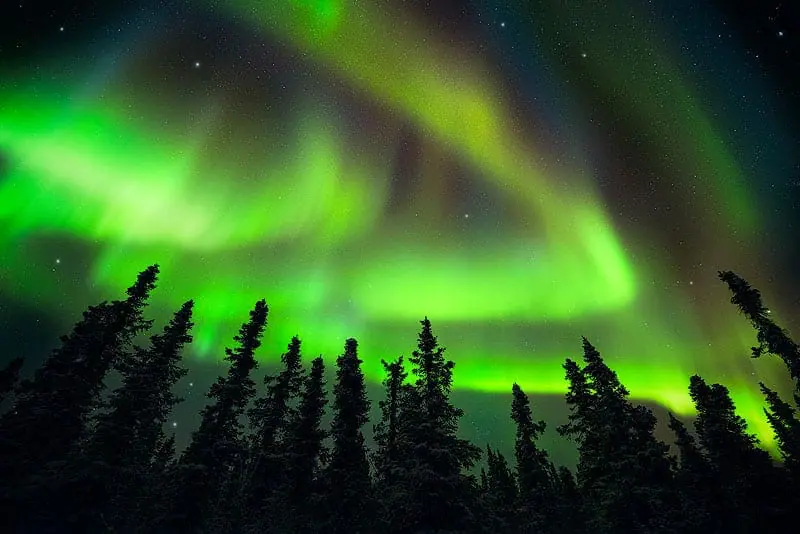This photograph depicts an outdoor setting at nighttime, seemingly capturing the northern lights. The scene is dominated by a strikingly lime green and dark gray sky, with areas of lighter green interspersed throughout. The bottom portion of the image is enveloped in darkness, showcasing the silhouettes of tall, pitch-black pine trees stretching from edge to edge. 

The trees' outlines are stark against the vibrant sky behind them, which transitions into varying shades of green and darker tones. As the eye moves upwards, the sky becomes increasingly dark, culminating in almost complete blackness at the top. Tiny stars are scattered throughout these darker areas, contributing to the nighttime ambiance.

The photograph, characterized by its blurred, old appearance, measures approximately five by five inches. It contains no identifying marks, annotations, objects, or persons, and lacks the presence of a moon. The overall scene, though not traditionally beautiful, offers a haunting glimpse of nature under a surreal, eerie light.